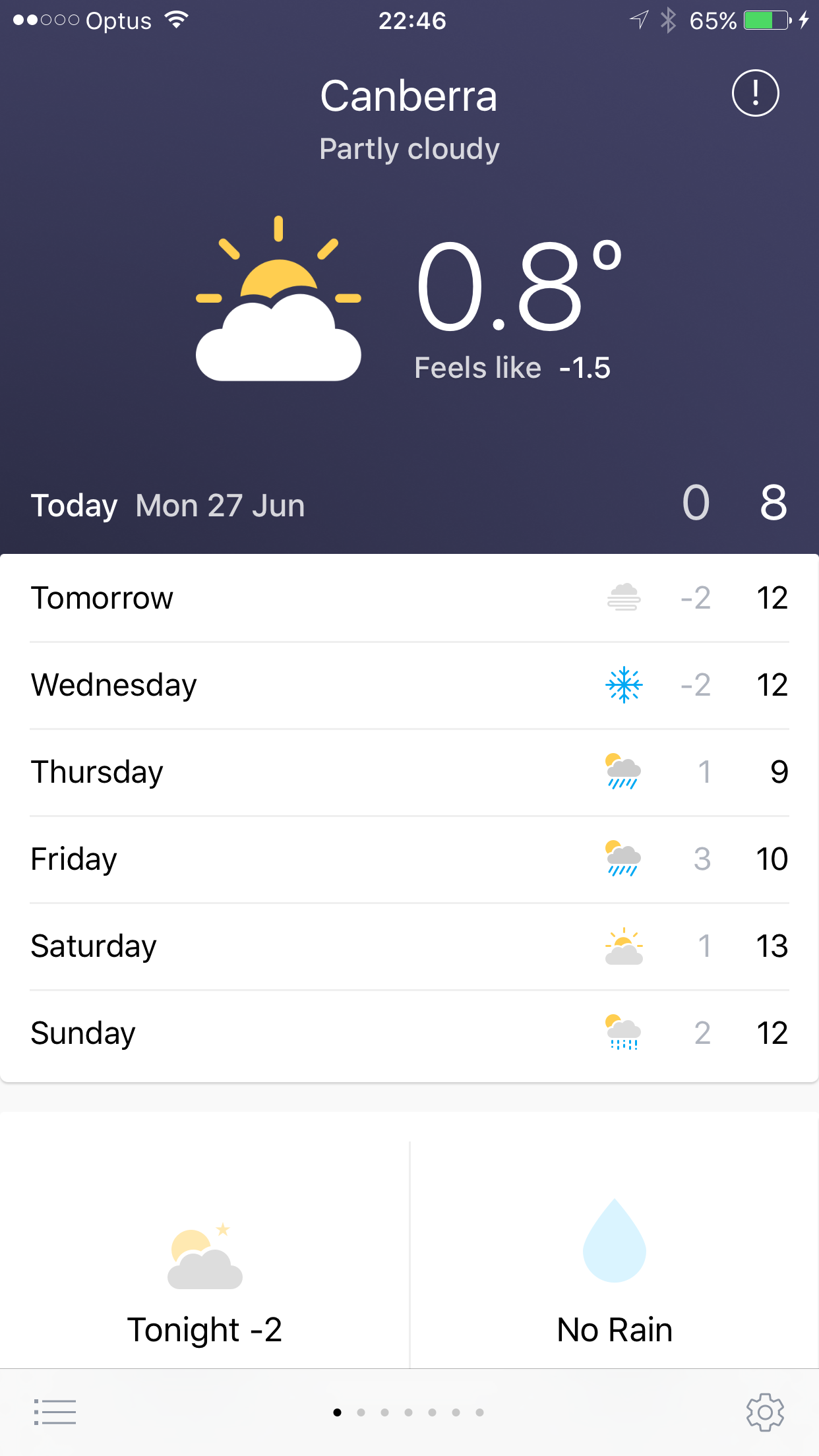The image is a screenshot from a mobile device displaying various status indicators at the top, including two circle-shaped carrier bars, the carrier name "Optus," enabled Wi-Fi, a location icon, an active Bluetooth connection, and a battery life of 65%. The time shown is 22:46. Below these indicators, there's a weather widget for Canberra displaying a partly cloudy condition with an icon featuring a sun partially obscured by a cloud. The widget reports a current temperature of 0.8°C, with a "feels like" temperature of -1.5°C. The date is noted as Monday, June 27th, and the forecast for the next day predicts a low of -2°C.